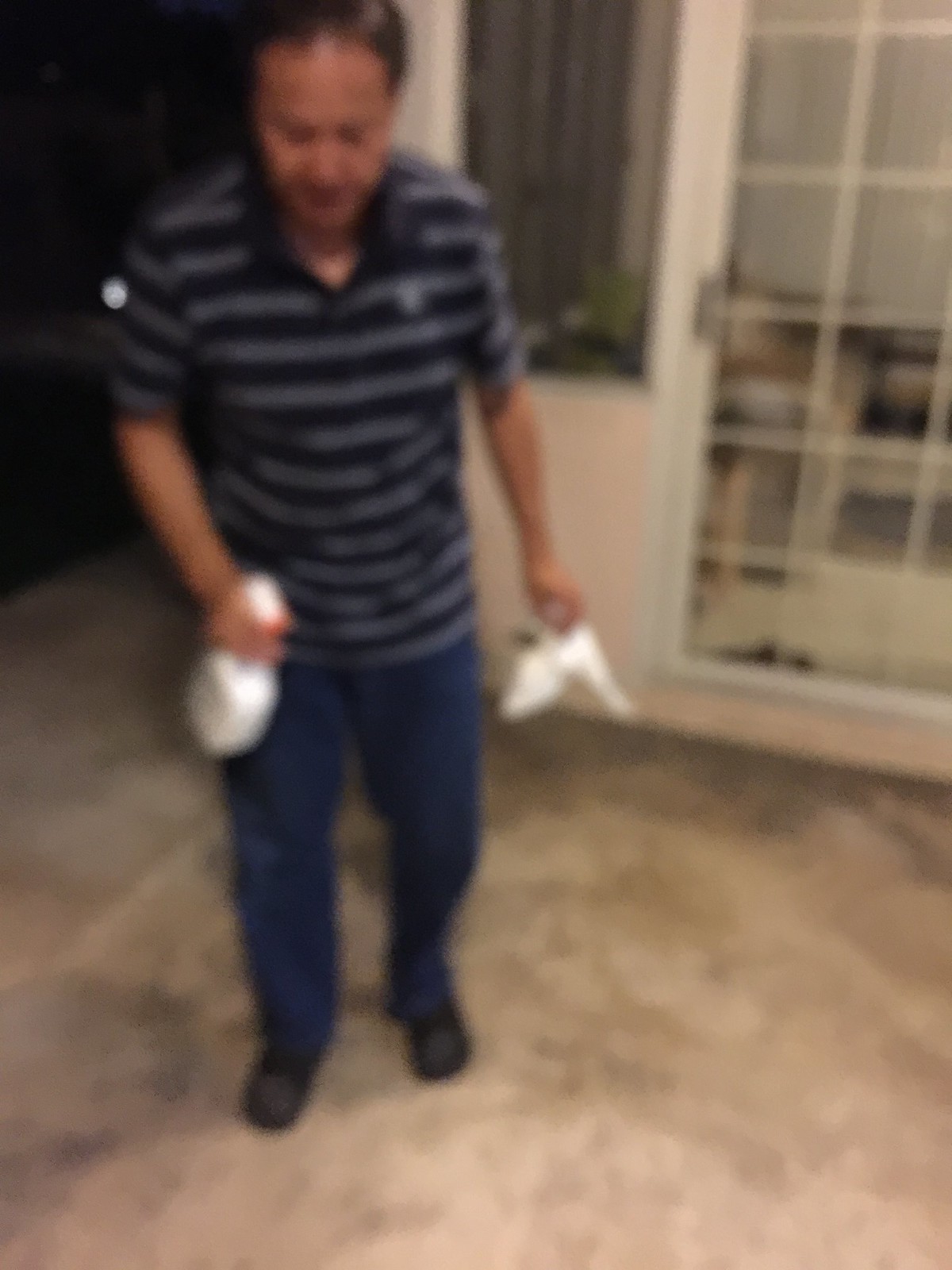This slightly blurry, vertically-oriented indoor photograph captures a middle-aged man, possibly in his 40s or 50s, holding cleaning supplies. He is standing on a granite-looking floor, clad in a short-sleeved black polo shirt with white horizontal stripes, dark blue jeans, and black shoes. In his left hand, he clutches a white paper towel while his right hand holds a white spray bottle with a nozzle. The man, whose head is slightly bowed, has thinning hair. Behind him, a pink wall features a window with a view of an opposite wall and a glass-paneled door to the right. The background to both his left and right sides appears dark, placing him in stark, contrast-focused center. The setting suggests he might be cleaning an area of the house.